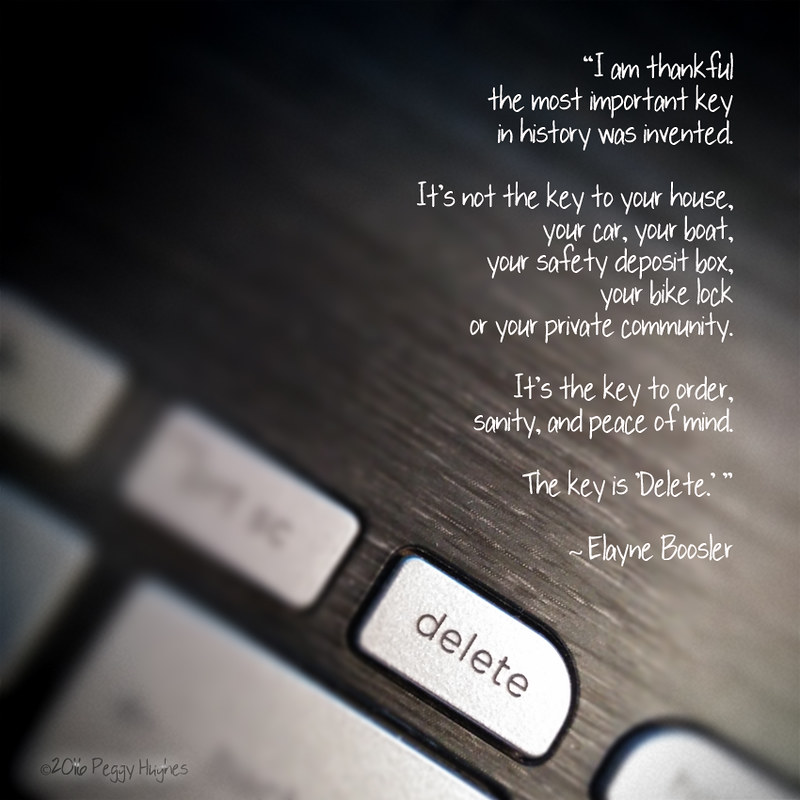The image shows a silver aluminum-finished laptop keyboard with an emphasis on the delete key, which is a silver oblong button. The surrounding keys are faded, drawing more attention to the delete key positioned towards the center bottom of the photo. The background features a wood grain texture in dark brown, providing a strong contrast to the sleek keyboard. In white text on the right side, the caption reads: 

"I am thankful the most important key in history was invented. It's not the key to your house, your car, your boat, your safety deposit box, your bike lock, or your private community. It's the key to order, sanity, and peace of mind. The key is 'delete.' - Elaine Booster."

The image appears to be digitally created, with some text on the buttons in black and a clear emphasis on the philosophical significance of the delete key.